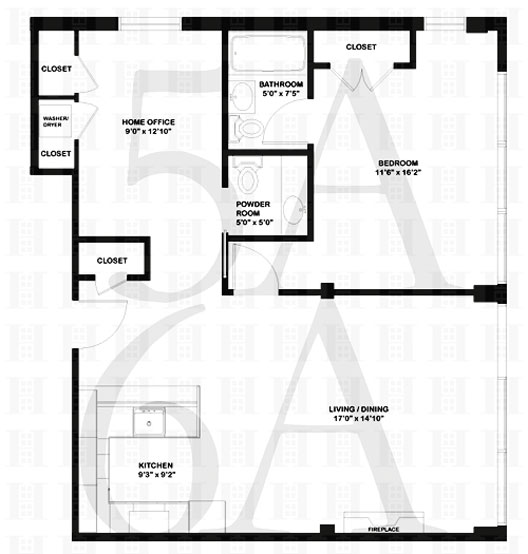This detailed floor plan is outlined in black and overlaid on a light gray background marked with "5A" at the top and "6A" at the bottom. 

At the upper section of the plan, there is a closet followed by a washing center, and then another closet. Adjacent to these storage areas is a home office measuring 9 feet by 12 feet 10 inches.

Continuing downward from the home office, there's another closet before reaching the kitchen. The kitchen itself is 9 feet 3 inches by 9 feet 2 inches. To the right of the kitchen lies the living and dining room area, which is spacious at 17 feet by 14 feet 10 inches and features a fireplace at the bottom.

From the home office going downward, there is a powder room measuring 5 feet by 5 feet. Moving upward from the living room, you will find a bedroom that is 11 feet 6 inches by 16 feet 2 inches, a bathroom that measures 5 feet by 7.5 feet, and an additional closet. The layout also includes an exit door towards the back.